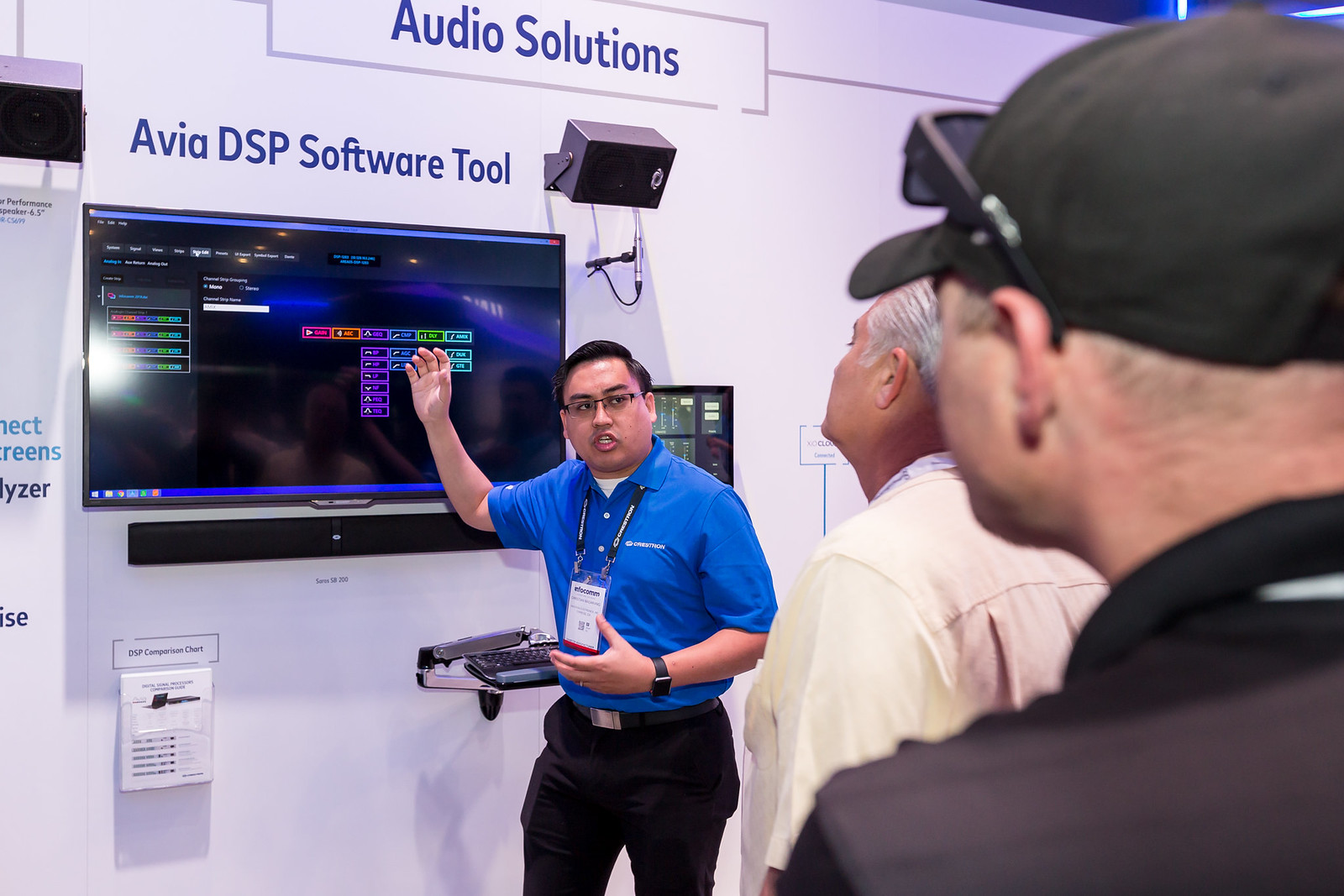In this photograph, which appears to be set in a modern indoor workplace or conference room, an Asian American man is giving a detailed presentation. He has short black hair and wears nerdy spectacles along with a lanyard and ID tag around his neck. Dressed in a blue polo shirt with white buttons and a black belt with a silver buckle, he stands before a large, very modern monitor displaying colorful boxes in shades of red, orange, purple, green, and various blues, complete with toolbars and icons. His right arm gesticulates towards the screen, emphasizing his points as he explains the Aviya DSP software tool, indicated in blue-purple lettering on the wall. Above the monitor, the words "Audio Solutions" are prominently displayed within a black-lined rectangle. Two other men attentively follow his presentation: one, perhaps white or Asian with gray hair in the background wearing a white shirt, and another, closer to the camera on the right, featuring a shaved buzz cut under a black baseball cap with perched sunglasses, dressed in a black and gray jacket. Behind the presenter, a vintage-styled window peeks out, adding to the room's ambiance. Below the monitor and a horizontal black line, there is a plastic case containing forms for perhaps self-serving purposes. Wires can be seen hanging from a wall-mounted, black-faced rectangular speaker in a gray frame bracketed to the upper section of the wall. The presenter's expression and posture suggest he is passionately explaining the software's benefits to his intrigued audience.